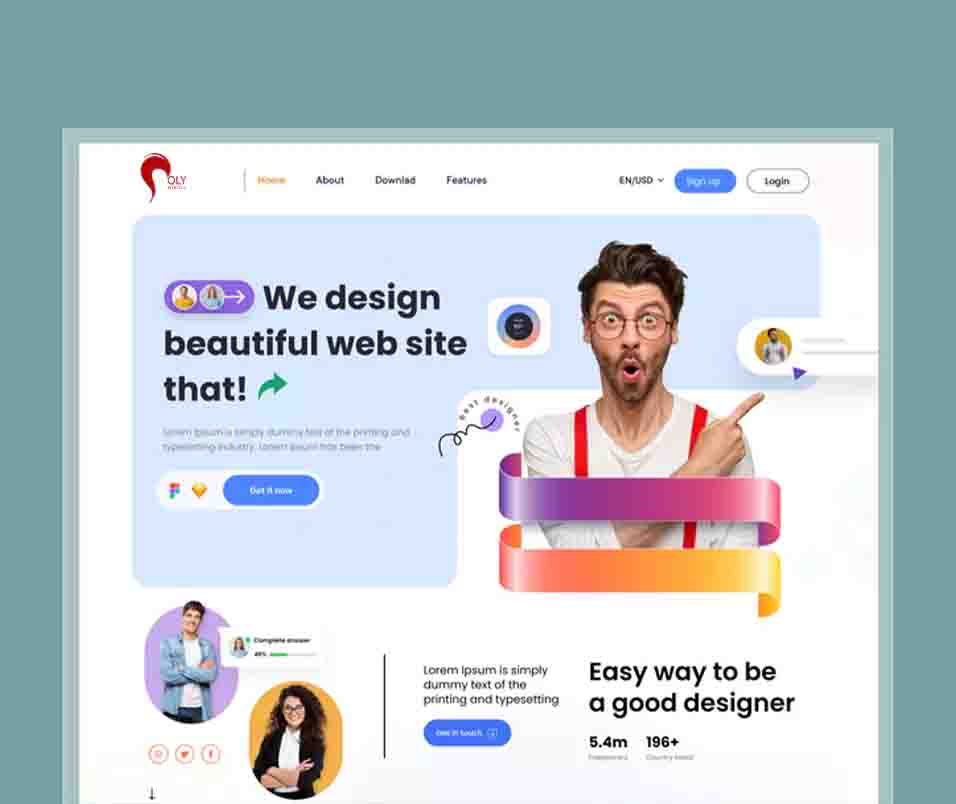The image features a green-colored border surrounding a detailed infographic. In the top left corner of the infographic is a logo that resembles red hair, accompanied by the text "Ollie." The central portion includes navigation options: Home, About, Download, and Features, with the Home button illuminated in orange. To the right of these options are the labels "EN" and "USD." A blue sign-up button with white text and a white login button with black text are positioned below the navigation. Below these buttons, there's a prominent picture of a man wearing red suspenders and a white long-sleeved shirt. He has glasses, a beard, and an open-mouthed, surprised expression, pointing upward with his right finger towards a box placed to the left of his shoulder. Adjacent to this image are the words, "We Designed Beautiful Website!" highlighted with a green arrow. At the bottom left of the infographic are two figures, and on the right side, the text reads, "Easy Way to Be a Good Designer."